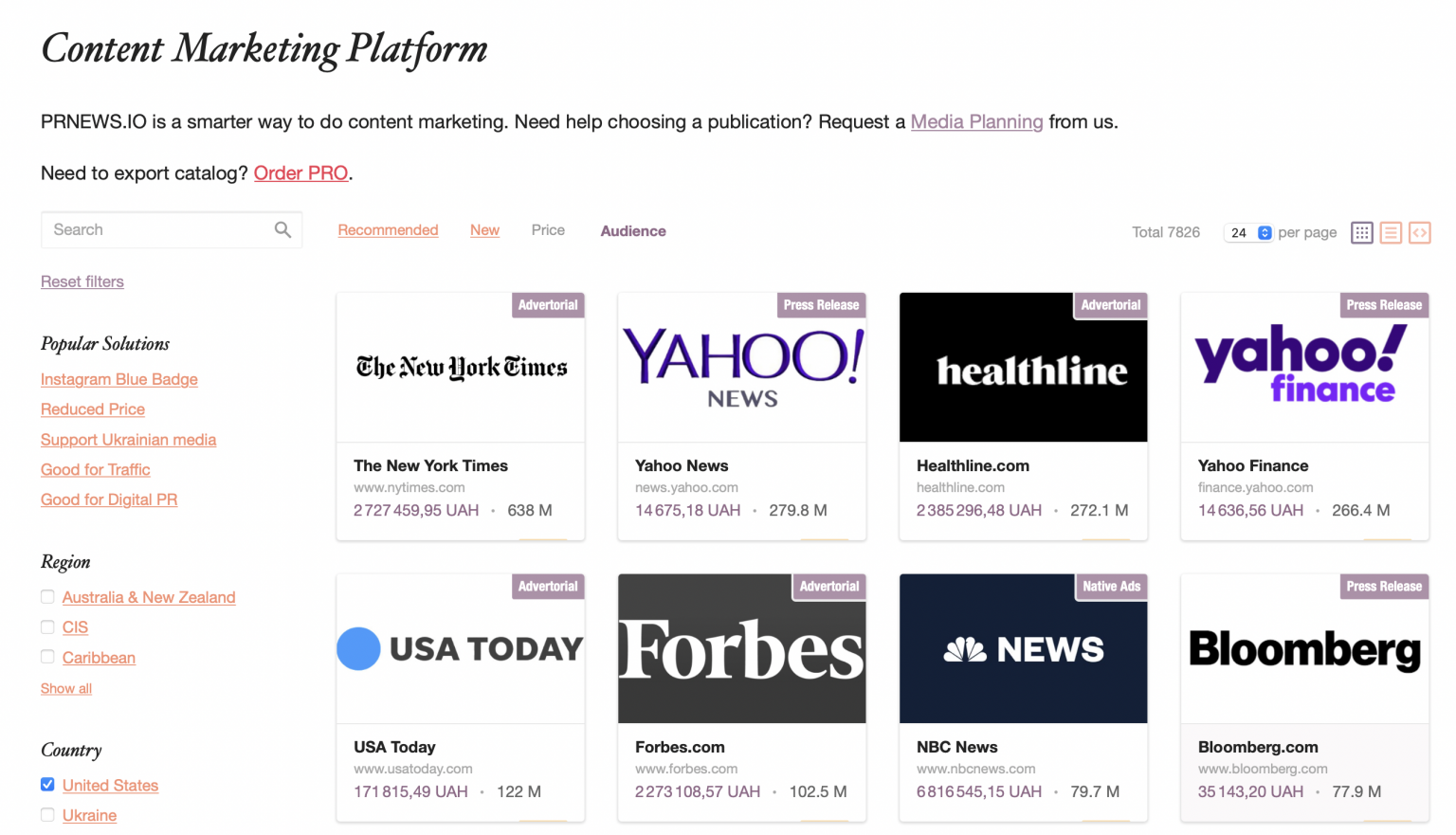This image showcases a content marketing platform named PREnews.io, presented in a landscape orientation against a clean, white background. The platform's interface is efficiently organized and features various tools for users. 

At the top left corner, the header "Content Marketing Platform" is elegantly scripted, followed by a subheading in standard black font stating, "PREnews.io is a smarter way to do content marketing." Below this, there's a highlighted and underlined prompt in purple: "Request immediate planning from us." 

Further down, the text "Need help choosing a publication? OrderPro" is mentioned, with "OrderPro" distinctively underlined in red font.

Beneath the header, an empty white search bar is positioned centrally, accompanied by filter options such as "Recommended" and "New" (underlined in red), and "Price" and "Audience" (with "Price" in gray and "Audience" in black). 

A Reset Filters button is situated directly below the search bar. Adjacent to this, three category headers in black font read "Popular Solutions," "Region," and "Country," each followed by a list of options in red links for users to select.

The main section of the interface showcases eight article thumbnails arranged in four columns and two rows. Featured publications include The New York Times, Yahoo News, Healthline, Yahoo Finance, USA Today, Forbes, NBC News, and Bloomberg. For each, users have the option to select either "Advertorial" or "Press Release."